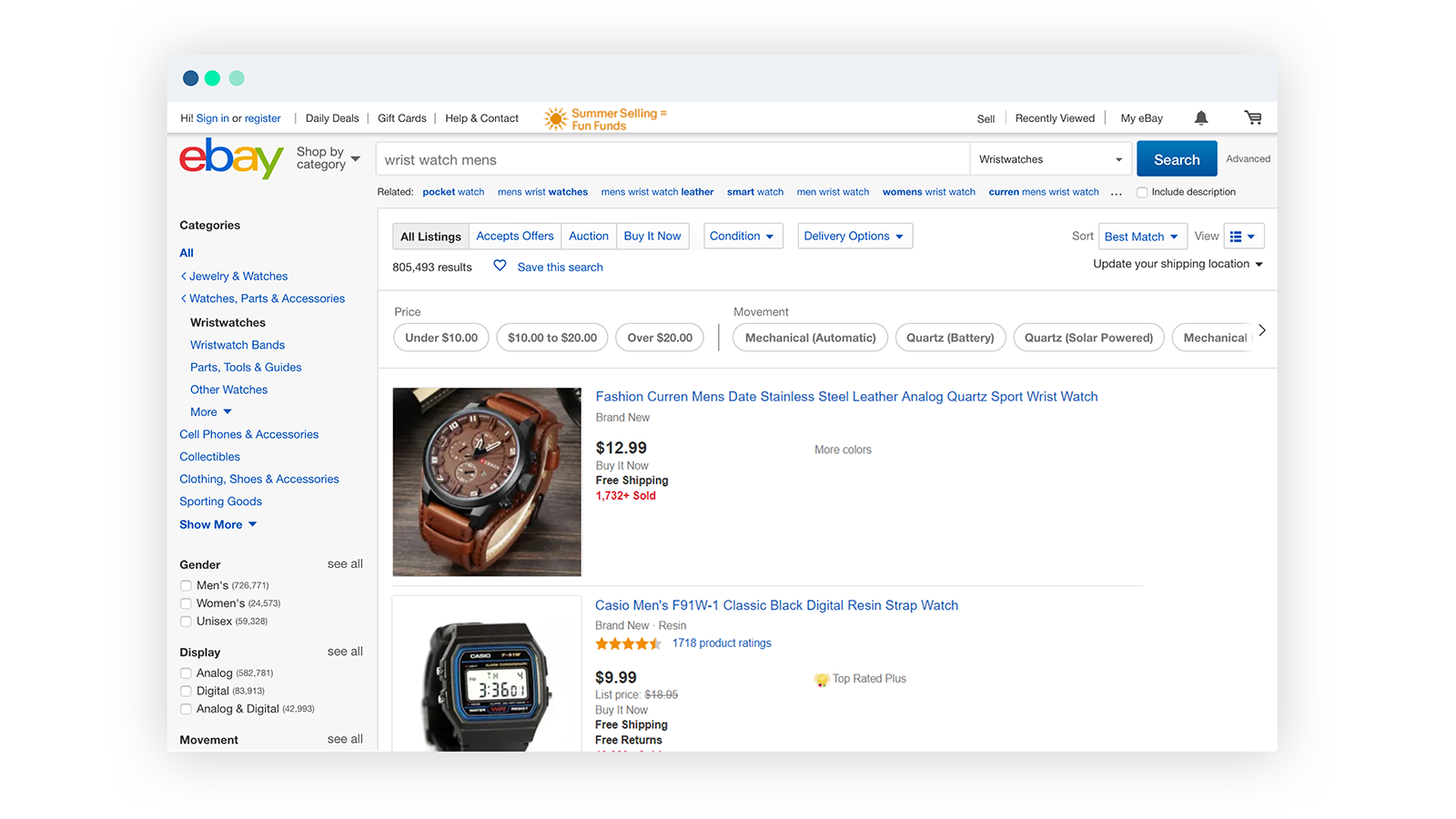The image showcases the homepage of a website, presumably eBay, characterized by a clean and structured layout. The top section of the page features a light gray background with a border, adorned with three colored circles: the first one is dark blue, the middle one is a light seafoam green, and the last one is a teal-blue seafoam green.

Beneath this section is a white banner containing hyperlinked text in blue, including "Hi! Sign in" and "Register," followed by additional links labeled "Daily Deals," "Gift Cards," "Help," and "Contact." An orange sun icon accompanies the text "Summer Selling Fun Finds."

To the right of this banner are more links labeled "Sell," "Recently Viewed," and "My eBay," along with icons for a notification bell and a shopping cart. The iconic eBay logo is positioned towards the left, composed of the letters 'e', 'b', 'a', and 'y' in red, blue, yellow, and green colors respectively.

Below this banner, an area designated for navigation features a "Shop by Category" option on the left, next to a search bar prefilled with the text "wristwatch men's." Related search suggestions such as "pocket watch," "men's wristwatches," "men's wristwatch leather," "smartwatch," and more are displayed.

The page displays various filters and sorting options including categories based on gender, display type, and movement. Central options highlighted include "All Listings," "Accept Offers," "Auction," "Buy It Now," conditions with a dropdown, and delivery options with another dropdown. Users can refine their search with dropdowns like "Store," "Best Match," "View," and update their shipping location.

Price filters listed are "Under $10," "$10 to $20," and "Over $20." Movement types are detailed as "Mechanical (Automatic)," "Quartz (Battery)," "Quartz (Solar Powered)," and "Mechanical," each with expandable options indicated by arrows.

Two product listings are prominently displayed: 
1. A men's fashion wristwatch with a stainless steel leather and analog quartz sport design priced at $299, brand new with a "Buy it Now" option and free shipping.
2. A Casio Men's F91W-1 Classic Black Digital Resin Strap Watch, brand new at $9.99, featuring free shipping and free returns.